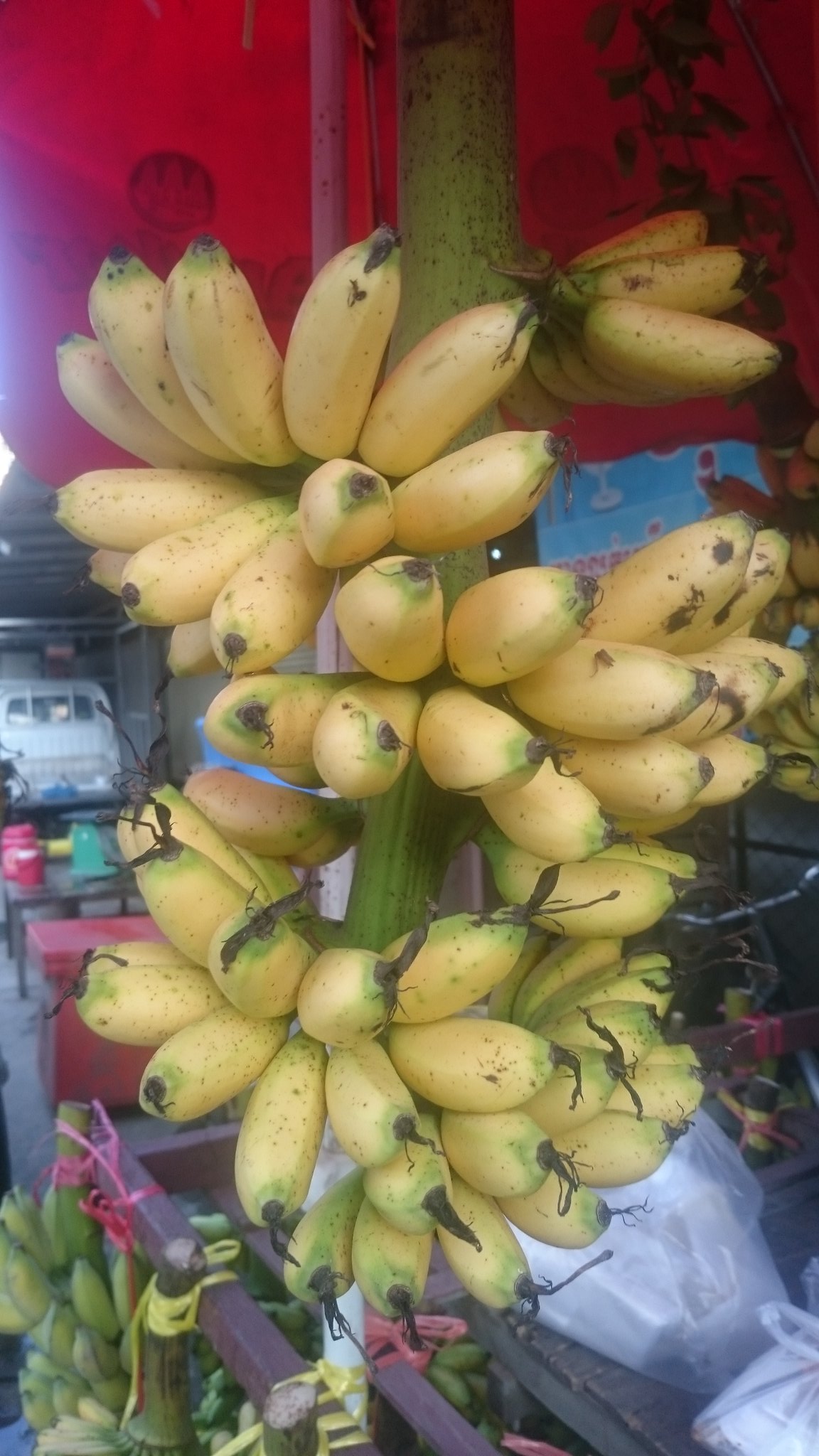This detailed photograph captures a bustling outdoor market scene, focusing closely on a large, green banana tree stalk that extends out of the frame. Bundles of medium-sized, yellow bananas, speckled with black dots and bruises, cluster densely along the stem. The bananas are either regular bananas or plantains, although their size renders them somewhat ambiguous between the two. In the lower left corner, greener bananas lie on the ground, hinting at varying stages of ripeness. The background reveals a vibrant market atmosphere with red tarps, street tables for dining, and assorted plastic bags, adding to the lively, everyday essence of the setting.